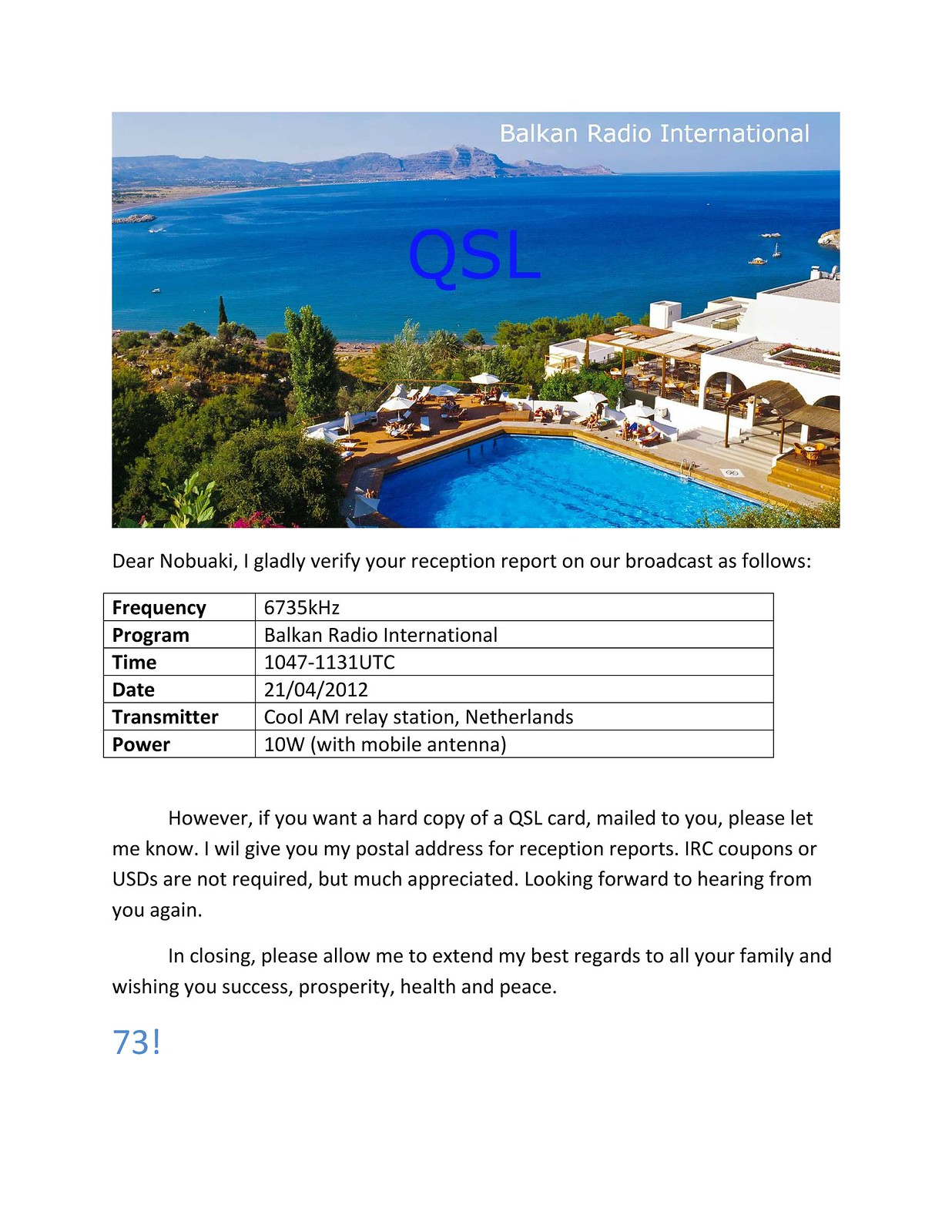The image is a detailed communication document sent to Nobuaki, formatted as a JPEG. At the top, there's a picturesque photograph of a luxurious beach resort. The resort features a large pool with blue water, surrounded by white sandstone buildings and umbrellas on the pool deck. The setting includes lush green trees and a distant view of mountains across the bay, suggesting a Mediterranean location. Superimposed on the photo, in blue letters over the ocean, is the text "QSL," while "Balkan Radio International" is written in white at the top right.

Below the photograph, the document transitions to a white background with text. It starts with a message: "Dear Nobuaki, I gladly verify your reception report on our broadcast as follows." This is followed by a detailed table listing the frequency, program, time, date, transmitter, and power of a radio broadcast:

- Frequency: 6735 kilohertz
- Program: Balkan Radio International
- Time: 1047, 1131 UTC
- Date: 2104, 2012
- Transmitter: CoolAM relay station, Netherlands
- Power: 10 watts with mobile antenna

The message continues, offering to mail a hard copy of the QSL card if requested, along with the postal address for reception reports, and noting that IRC coupons or USDs are appreciated but not required. It closes with well-wishes for Nobuaki's family and success, prosperity, health, and peace, and ends with "73!" in blue at the bottom left.

The overall layout presents a blend of visual and textual elements, suggesting it might be an internal communication or notification from the radio station, encapsulating various details about the transmission and the station's gratitude for the reception report.